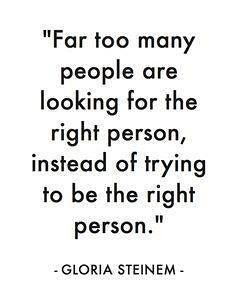The image features an inspirational quote by Gloria Steinem centered on a stark, white background. The quote, presented in bold black text, is meticulously formatted into seven lines: "Far too many / people are / looking for the / right person / instead of trying / to be the right / person." Below the quote, the author's name, "GLORIA STEINEM," is displayed in all capital letters with a dash on either side. The minimalist design, which includes no other objects or text, creates a floating effect that emphasizes the motivational message, making it a typical example of content shared on social media platforms like Pinterest.